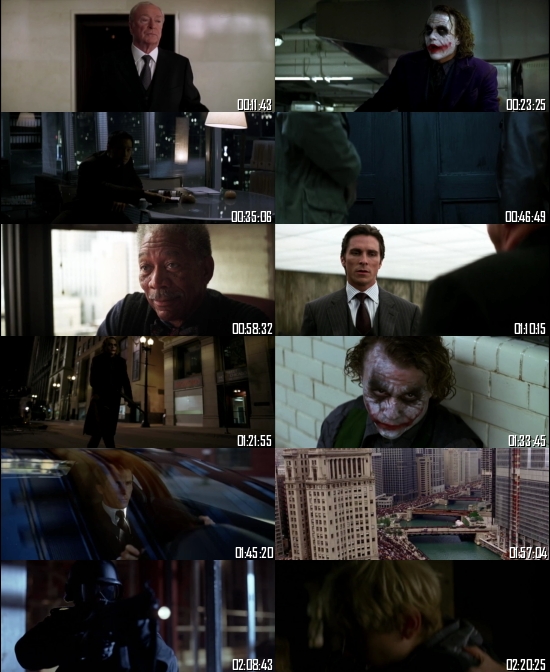This image is a detailed collage of twelve movie stills from a Batman movie, showcasing various scenes featuring The Joker, who appears notably at timestamps 23:25 and 33:45. The collage is arranged vertically into two columns of six images each. Each still is marked with a six-digit timestamp format (hh:mm:ss). The Joker, dressed in his iconic purple suit jacket, is seen in a couple of these screenshots, one of which shows him leaning against a green brick wall. The scenes capture both indoor and outdoor settings, including an apartment, city streets, and the exterior of buildings. Various characters make appearances, including other male characters, an older man in a suit at the top right, a black man, and someone wearing a hat. The diverse settings also include someone driving a car and a cityscape, providing a comprehensive visual representation of different moments from the film.